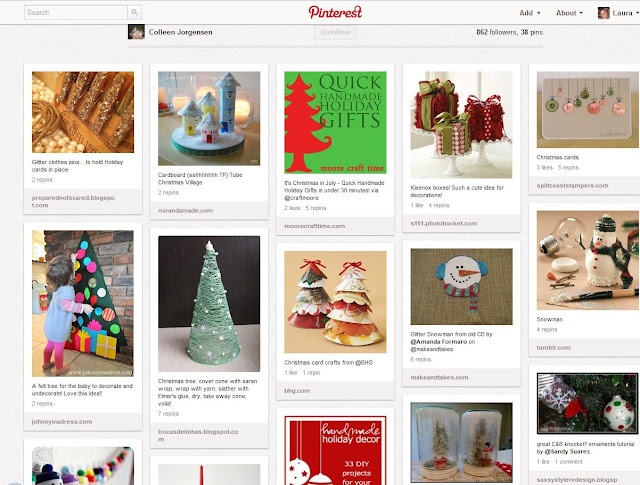This image appears to be the Pinterest homepage for the user "Colleen Jensen" or "George Jorgenson" (spelled J-o-r-g-e-n-s-e-n), featuring a profile named Laura. The page illustrates a button to unfollow this user, who has 862 followers and 38 pins.

On the right-hand side of the image, there are options such as an "Add" button and a dropdown menu featuring Laura's profile photo. Below these elements, there is a line separating the profile details from the series of pins.

The pins are arranged in three rows, with the first two rows fully visible and the third row partially cut off. In the first row, there are five pins:
1. A glitter-covered clothespin meant for holding holiday cards in place.
2. A cardboard Christmas village.
3. Quick, handmade holiday gifts.
4. Decorations made using Kleenex boxes, although the resolution of the image makes this pin hard to read.
5. A cute idea for using Christmas cards as decorations.

The second row features:
1. A felt tree designed for a baby to decorate.
2. A DIY Christmas tree made from crates wrapped in saran wrap, resembling a Christmas tree structure.

Each pin displays images and descriptions that hint at creative holiday projects and decorations.